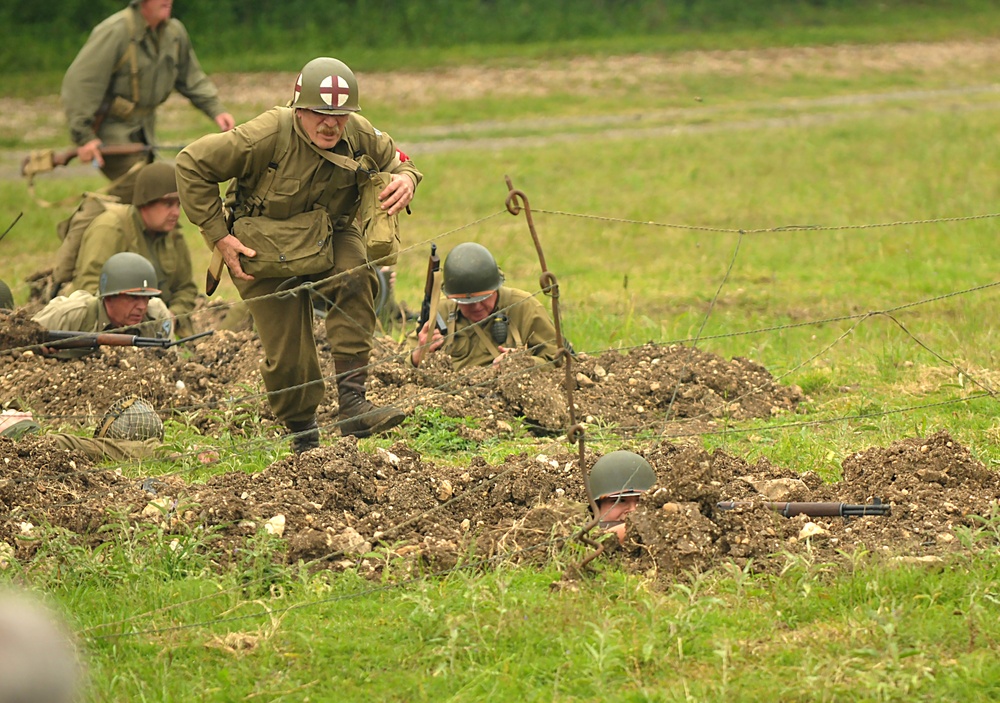The photograph captures a detailed reenactment of a World War I trench battle, situated in a large, grassy field under overcast skies. The background reveals several soldiers in period-appropriate green fatigues and round, heavy metal helmets. A row of fence posts with ropes and twisted iron rods forms a makeshift barrier. In the middle background, a soldier stands holding his rifle, while another crouches nearby. Trenches and foxholes are scattered across the field, offering cover for the reenactors. In the foreground, a gunner aims his rifle ahead, lying prone on a mound of dirt. Approaching swiftly from behind is a medic, distinguishable by the red cross emblem on his helmet and armband, carrying two bags of equipment, ready to assist the gunner. Additional soldiers in the distance are either holding their rifles or crouching for cover, simulating the chaos and strategy of trench warfare. The scene is meticulously set with fake weapons and authentic looking props, underscoring the dedication to historical accuracy typical of reenactments.